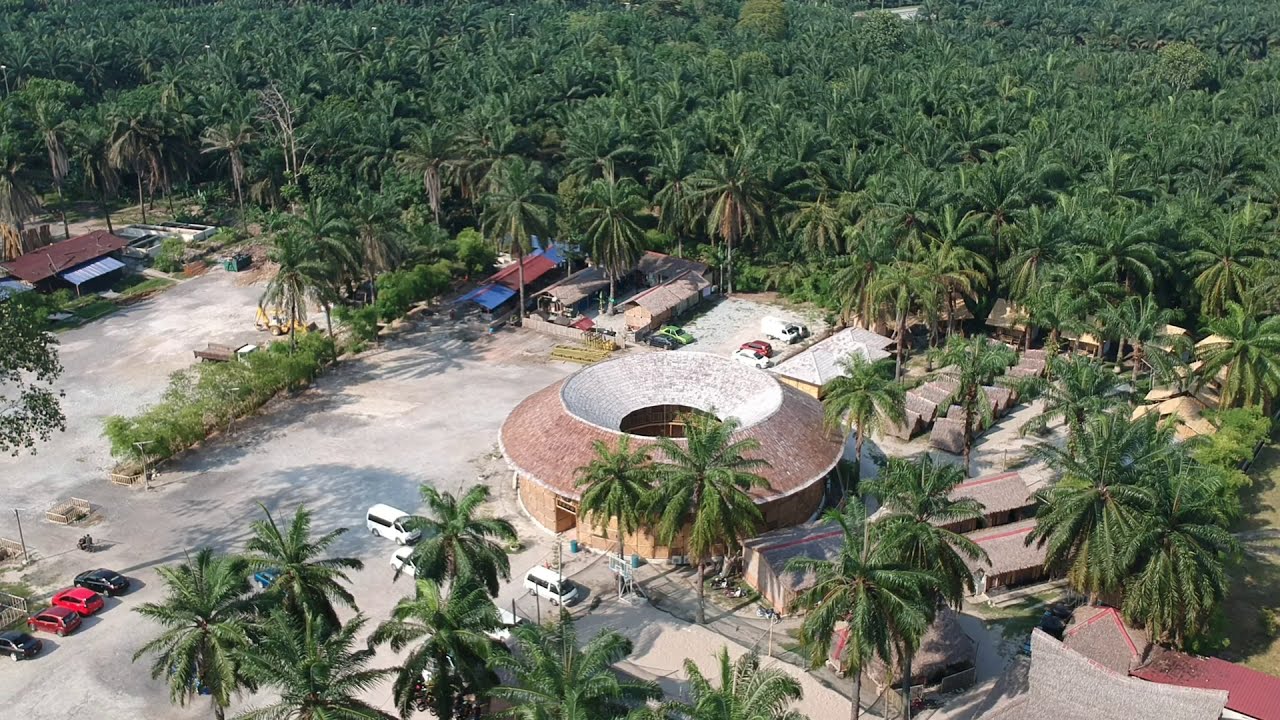This aerial photograph depicts a horizontally aligned rectangular image dominated by a dense canopy of green palm trees occupying the upper half. The center focus is a circular stone building with a red roof, featuring a hole cut out at the top and white interior walls. Surrounded by these trees, the building might be a part of a tourist destination or resort. In front of this structure, several white shuttle vans are parked, alongside a cluster of vehicles located in the lower left-hand corner: a black, a red, a dark red, and a gray car. Scattered throughout the bottom third of the image are additional palm trees. Towards the top left corner, there’s a structure with a brown roof and a smaller white awning, while more small, low structures with brown roofs are visible behind the circular building. The photograph encapsulates a lush, verdant landscape with carefully placed architectural and vehicular elements, all viewed from an elevated perspective.